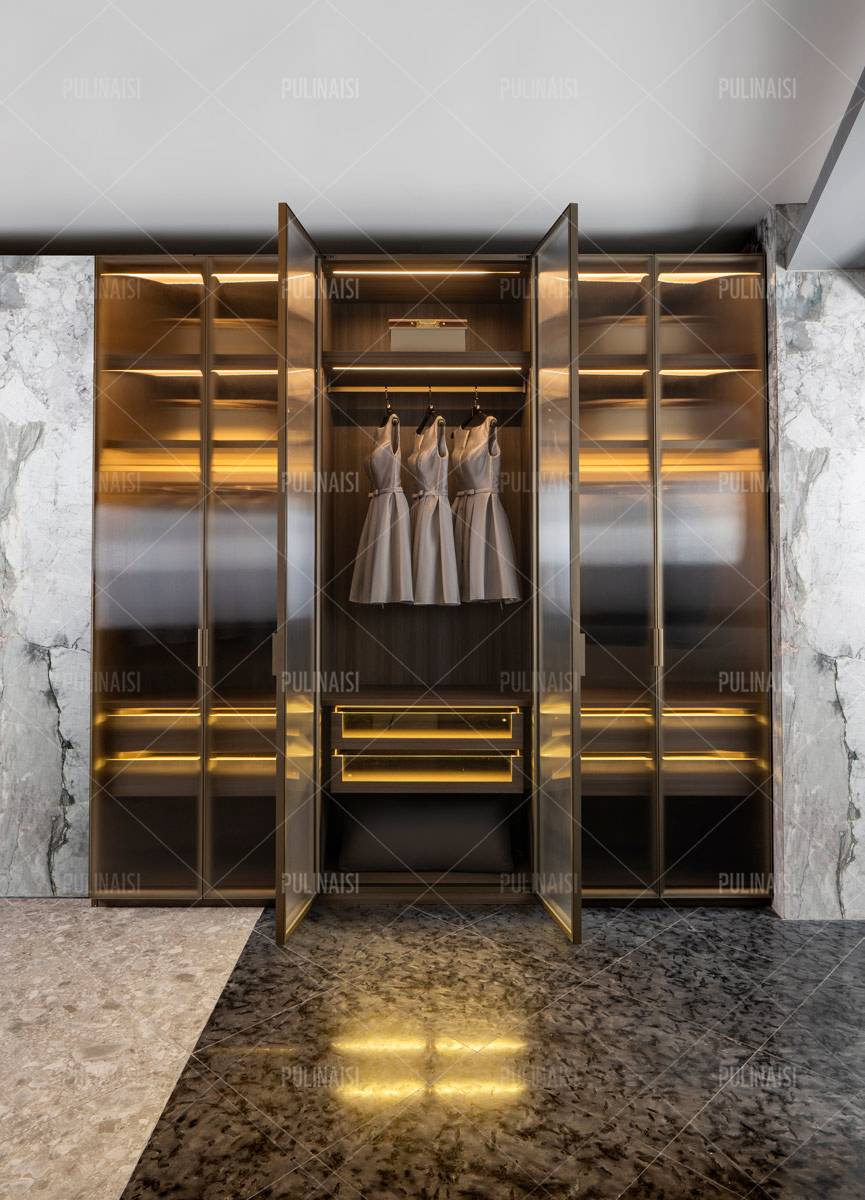This photograph showcases a luxurious, high-end closet or showroom interior, captured in portrait mode. The scene features a meticulously designed space framed by three glass panels, possibly metallic with a golden hue. The interior is elegantly illuminated, highlighting the intricate design. The closet is segmented into three compartments, each equipped with hanging spaces, drawers, and shelves. 

Three silvery-beige dresses, potentially bridesmaid dresses, hang prominently in the center, adding a touch of sophistication. The flooring is a stunning display of dark and light stones, transitioning from dark marble to white marble, contributing to the opulent atmosphere. The surrounding walls are adorned with marble, possibly granite, enhancing the overall luxurious aesthetic. The ceiling is gray, completing the refined look of the space.

This polished and stylish interior is identified by a watermark with the label "Polnicei," indicating its upscale nature and stock photo origins.